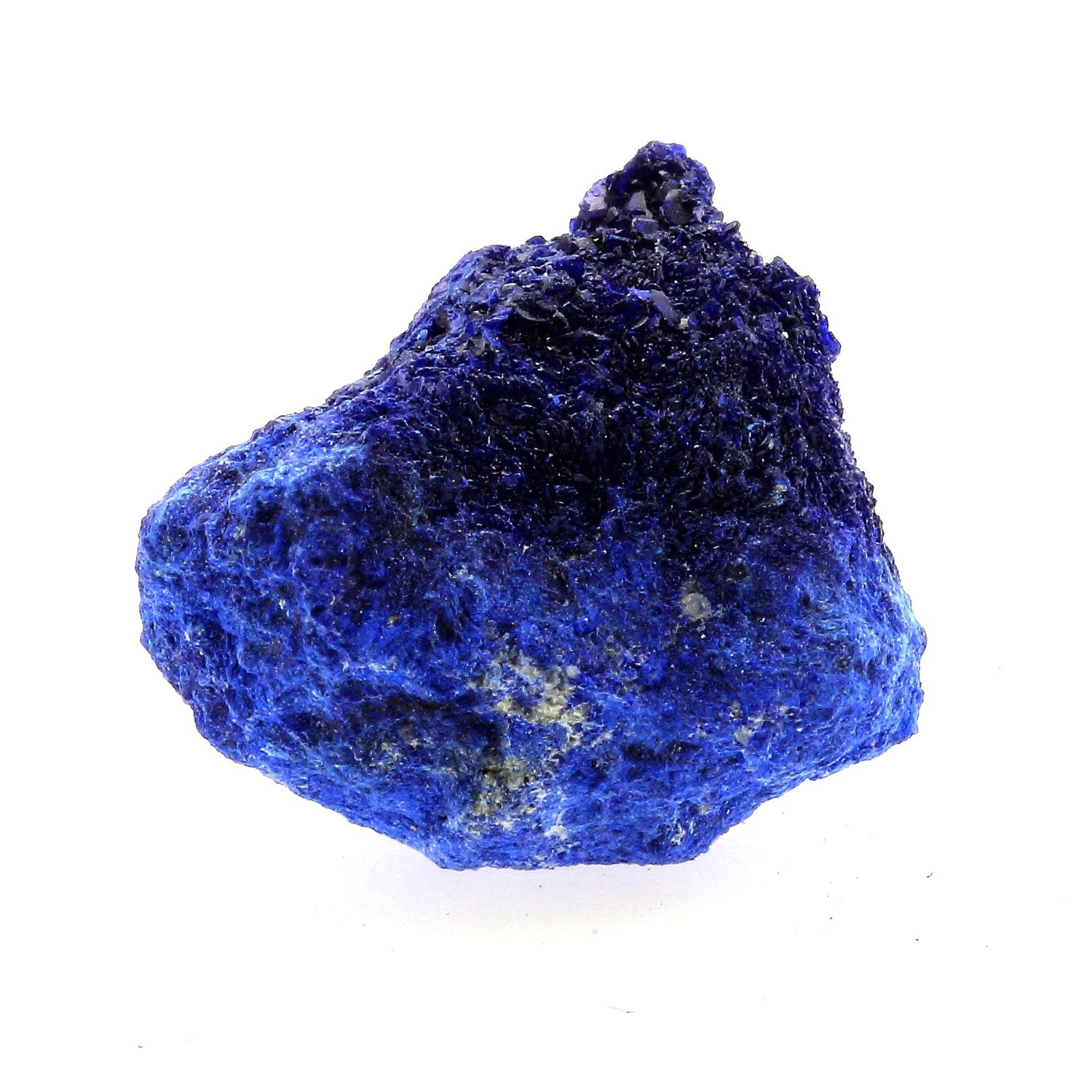This vertical image showcases a striking blue mineral or gemstone set against a white background. The rock features various hues of blue, transitioning from a lighter blue at the base adorned with white veins, to a darker blue, almost black, at the pointed and jagged top. The mineral's shape is irregular, with distinct cylinders or columns protruding, giving it a rough, porous appearance. The top is especially jagged and sharply defined, tapering to a point, while the bottom is smoother and more cylindrical. The white accents are primarily concentrated near the lighter blue sections at the bottom, adding a stark contrast to the dominant blue tones. Overall, this detailed and vibrant gemstone captures the eye with its multifaceted blue shades and rugged texture.